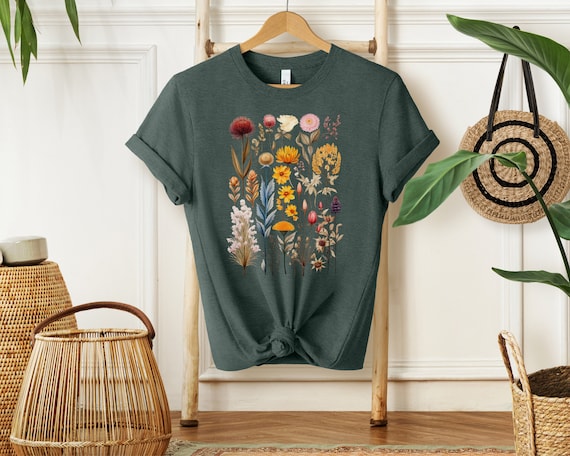In this image, a dark grey t-shirt with short, cuffed sleeves hangs on a wooden hanger from a rustic wooden ladder. The shirt features an intricate screen-printed design of various flowers—including red, white, blue, orange, yellow, purple, pink, and gold—neatly arranged in a rectangular pattern on the chest. The bottom of the shirt is stylishly knotted. Surrounding the shirt, there are several wicker baskets and a round woven purse hanging next to it. Greenery is also present, with some plants in wicker planters visible to the left and to the right, partially obscured by the frame. The background shows details of an off-white wall and a wooden parquet floor, completing a cozy, earthy aesthetic.